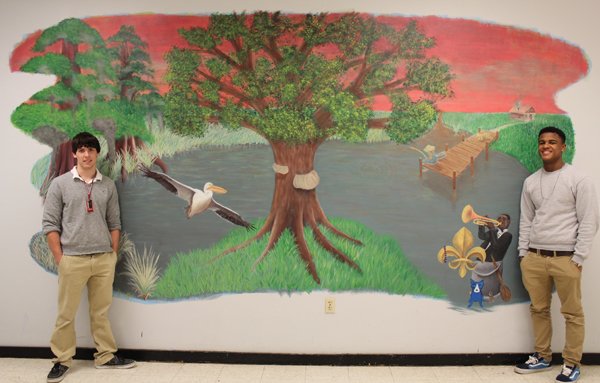The image captures two young gentlemen standing at both ends of a vibrant mural painted on a wall. The mural features a brown tree with lush green leaves, standing prominently in a grassy area surrounded by a body of water. Within this tranquil scene, a white stork or gull flies on the left side. Toward the right side of the mural, a gentleman, elegantly dressed in a tuxedo, plays a horn while standing in a boat with a paddle. Additional details include a dock in the background with a person possibly fishing, and a house nestled among other trees in the distance under a distinctive pinkish-red sky. Central to the mural is a symbol resembling a saint's insignia and a gray satchel with an oar. In the foreground, the two gentlemen appear happy as they pose. The gentleman on the right is Black, wearing a gray crew neck sweater, khaki pants, blue and black Vans Old Skool shoes, and a chain around his neck. On the left stands a white gentleman with dark hair styled in a bowl cut, dressed in a gray long-sleeved shirt over a white collared shirt, khaki pants, and gray shoes, wearing a lanyard around his neck. Both individuals give an impression of either being students on a trip or the artists of the mural.